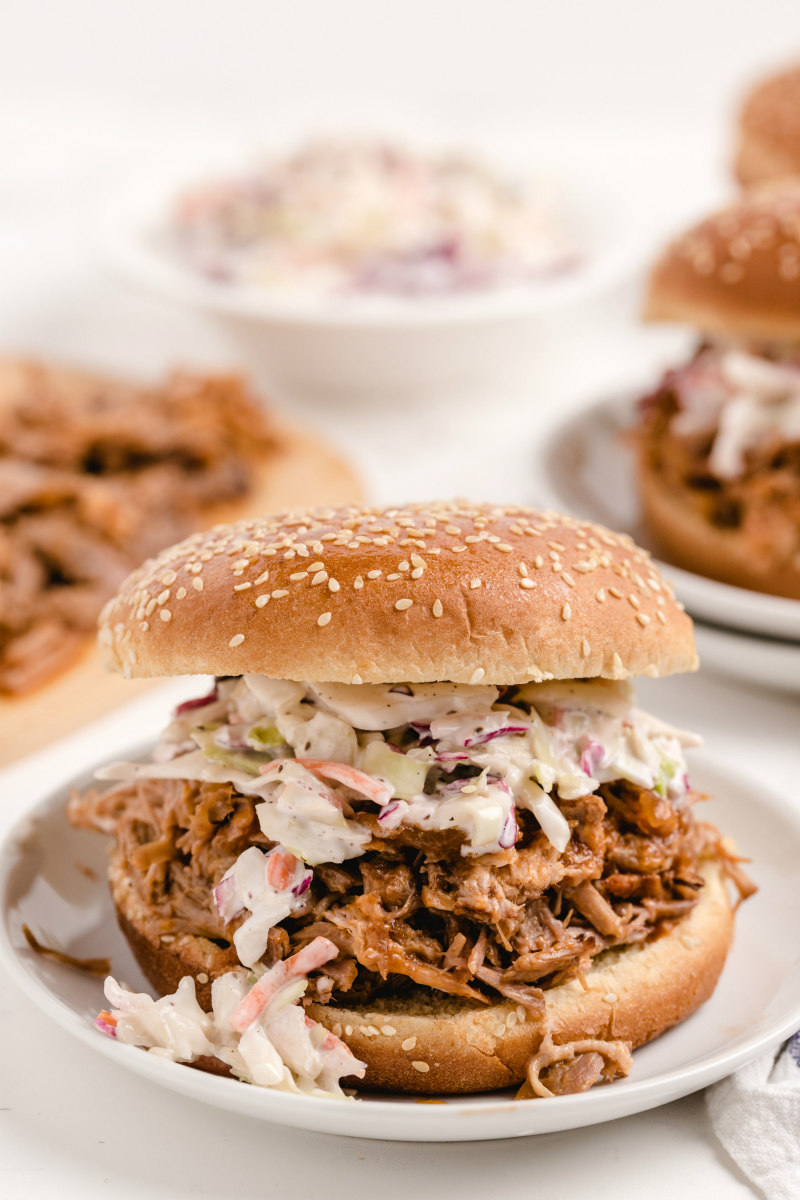The image showcases a delectable pulled pork sandwich, prominently positioned in the center of the photo on a white plate. The sandwich features a large sesame seed bun, generously filled with a layer of light and tangy coleslaw on top of a substantial portion of reddish-brown pulled pork. The close-up highlights the textures and colors vividly: the orange-ish brown and light green of the coleslaw, contrasting with the deep, rich hue of the pulled pork, all encased in the light brown bun speckled with white sesame seeds.

Surrounding the main sandwich, slightly out of focus, are more sandwiches and a tray of meat situated towards the left middle of the image, with additional burgers placed on the right middle. The top middle of the image shows more coleslaw, adding to the overall visual feast. The setting, bathed in warm tones of orange, light purple, and black, enhances the appetizing appeal of the scene. The detailed focus on the front sandwich emphasizes its mouth-watering look, making it the centerpiece of this culinary display.